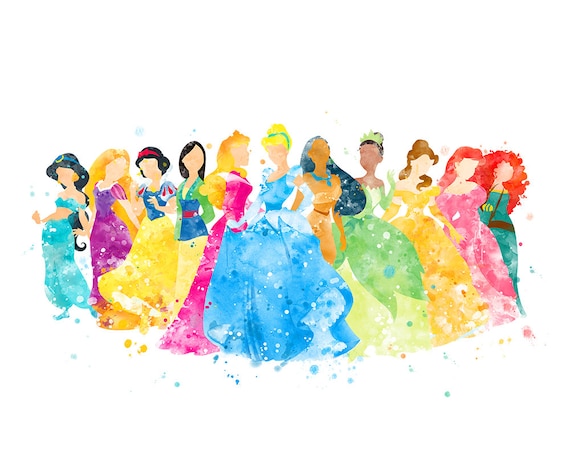The illustration depicts Disney princesses in a Neiman-style painting, characterized by a watercolor-like quality with imperfect details and no faces. The princesses form a V-shape centered around Cinderella, with each princess angled towards her. The vibrant, colored shadows and abundant use of white enhance the dreamy aesthetic. To the left of Cinderella are Sleeping Beauty, Mulan, Snow White, Rapunzel, and Jasmine, all adorned in their iconic dresses. To the right are Pocahontas, Tiana, Belle, Ariel, and Merida, each vividly dressed as they are famously recognized. The rightmost figure, Merida, is distinguished by her voluminous red hair and green dress with a brown belt.